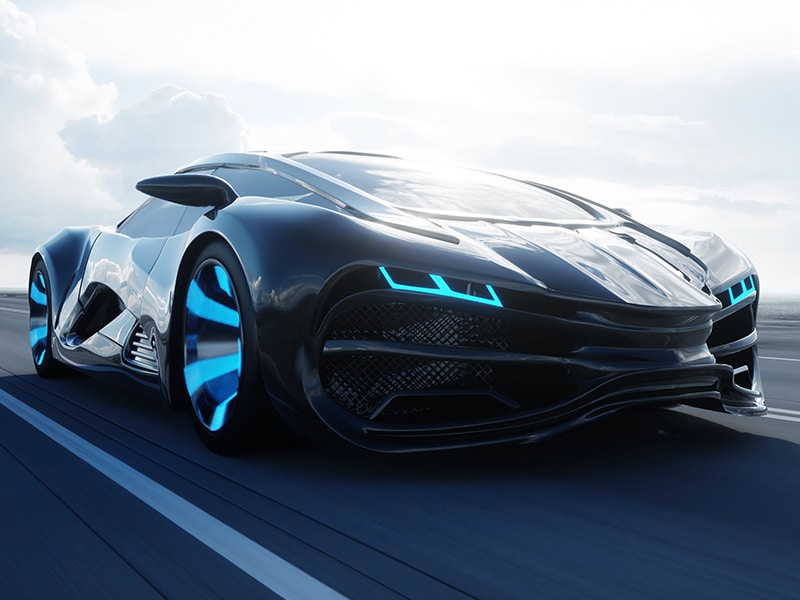The image depicts a highly futuristic, AI-generated car set against a backdrop of a bright blue sky adorned with white, fluffy clouds and sun glare. The car itself sports an unconventional and sleek design, with an overall dark blue hue. It features electric blue accents on its taillights and headlights, along with matching electric blue collars on the wheels. The car's structure includes spear-shaped side mirrors that angle downward, a unique wave-like rear pattern, and a massive glass top extending across its center, essentially replacing a traditional windshield. The car's grille, outlined in blue square lights, gives it an aggressive look. Its large wheels are equipped with light blue electric spokes, adding to its cutting-edge appearance. The road it is on appears surreal, enhancing the otherworldly feel. This narrow, seemingly impractical two-seater vehicle also hints at design elements that could allow its doors to open similarly to those of a DeLorean. Despite some suspicious rendering irregularities that suggest AI generation, such as the mismatched front perspectives, the car's overall aesthetic is unmistakably futuristic.